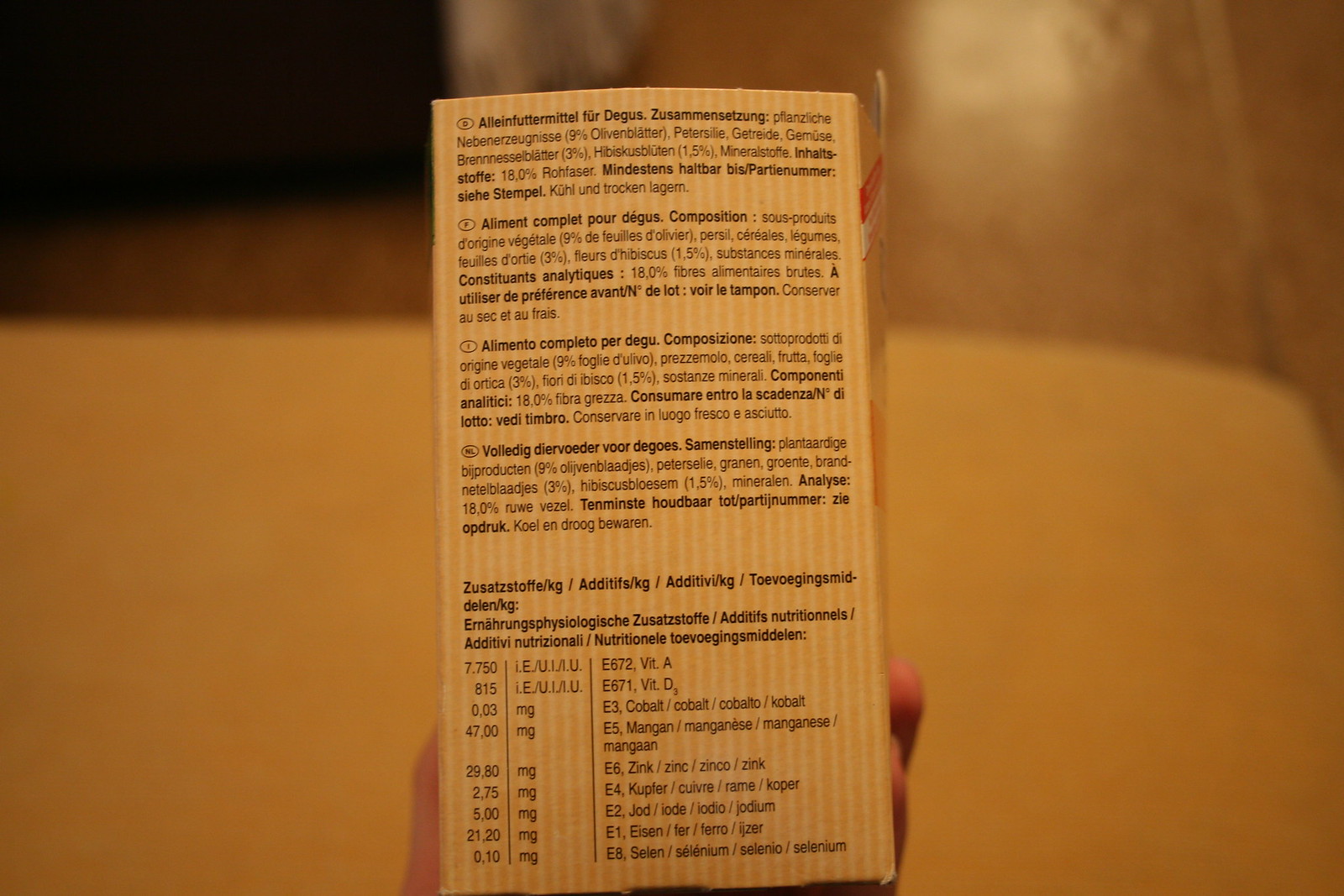The image showcases the back of a box adorned with foreign, non-English text. The written information is arranged in four distinct points, each accompanied by a paragraph. Below these paragraphs, there is a chart, seemingly related to the text above. The content suggests that the box might belong to a supplement or similar product.

In the image, a hand partially grips the box, with visible fingers on both the left and right edges. The lower part of the image features a slightly blurry area, possibly indicating a tabletop. The upper section reveals a tiled floor, while the top left corner of the image includes a black object, the nature of which is unclear.